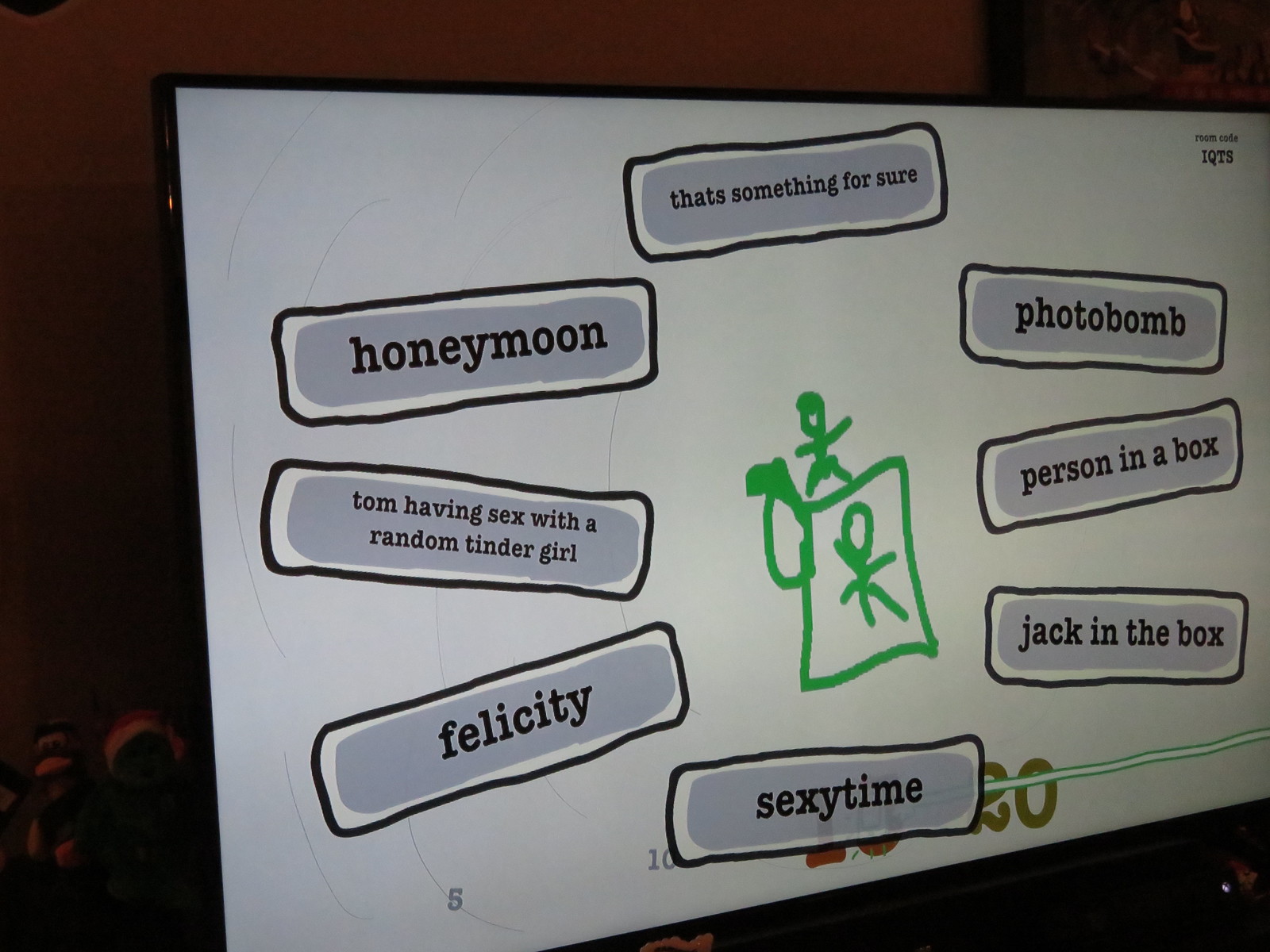In the image, a television screen displays a snapshot from the party video game "Jackbox." The screen features a solid white background with a central drawing, likely made using markers or digitally mimicking that effect, depicting stick figures—one lying down, seemingly on a bed, and another standing nearby. Surrounding this central illustration are several rectangular boxes outlined in black with gray interiors, each containing black text. At the top, one rectangle reads "That's something for sure." Additional text boxes encircle the drawing in a somewhat circular arrangement, with captions such as "Sexy Time," "Honeymoon," "Tom Having Sex with a Random Tinder Girl," "Felicity," "Photo Bomb," "Person in a Box," and "Jack in the Box." The setup appears to be interactive, as indicated by the room code "IQTS" in the top right corner, facilitating game participation via smartphones. The screen's background comprises a dark, brownish-black hue with subtle lighting effects.